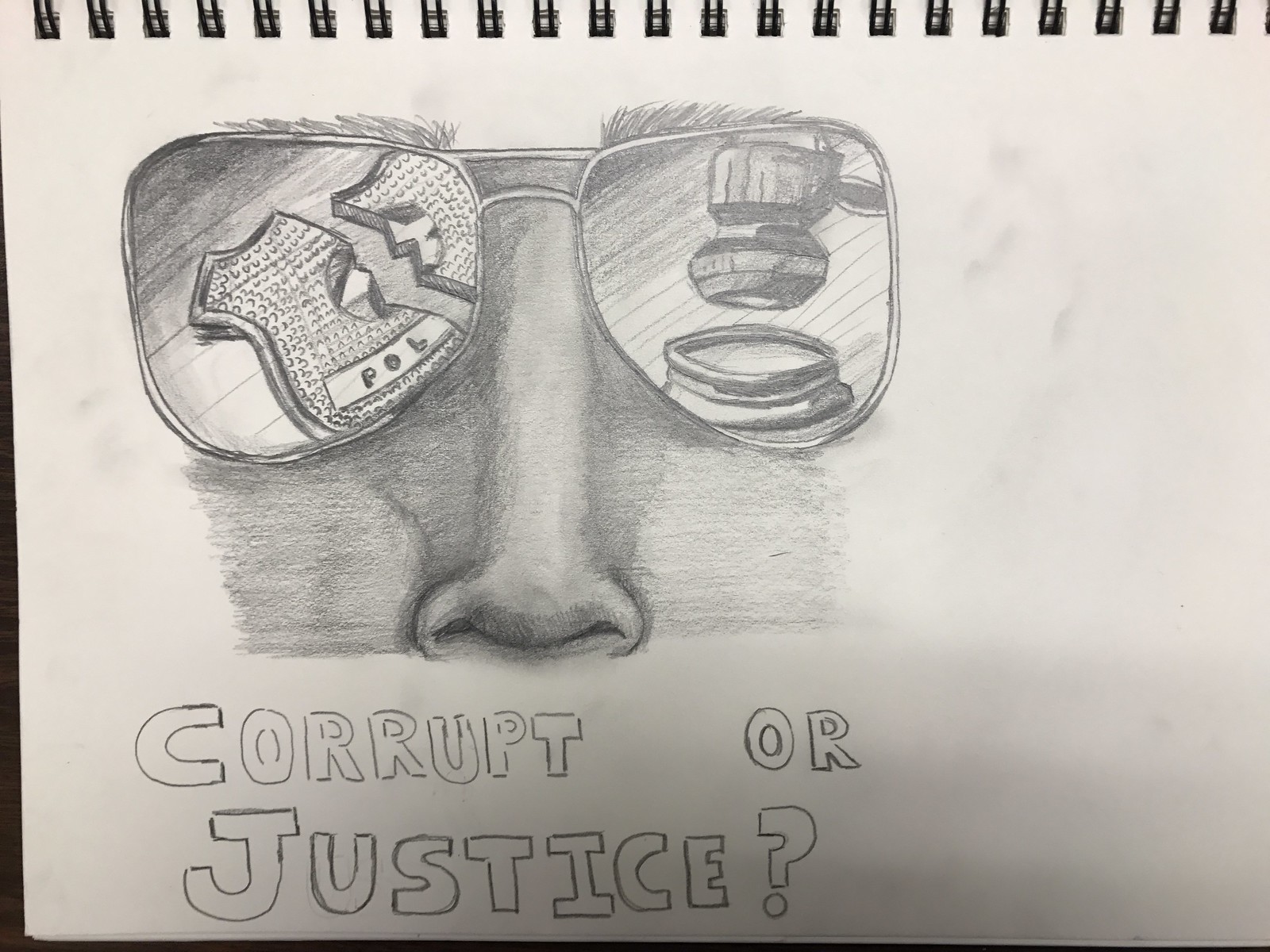A detailed pencil sketch on a white page of a spiral-bound sketchbook features a partial face with prominent eyebrows, a nose shaded to accentuate the nostrils, and reflective aviator sunglasses. In the left lens of the sunglasses, there's a detailed reflection of a police badge broken in half with jagged edges, showing the letters "P.O.L." On the right lens, there's a depiction of a judge's gavel poised to strike. Below this intricate drawing, in bold block letters, is the phrase "CORRUPT OR JUSTICE?" emphasizing the dichotomy. This sketch, likely a student's work, showcases varied shading techniques and slight proportional imbalances that convey a critical social commentary.